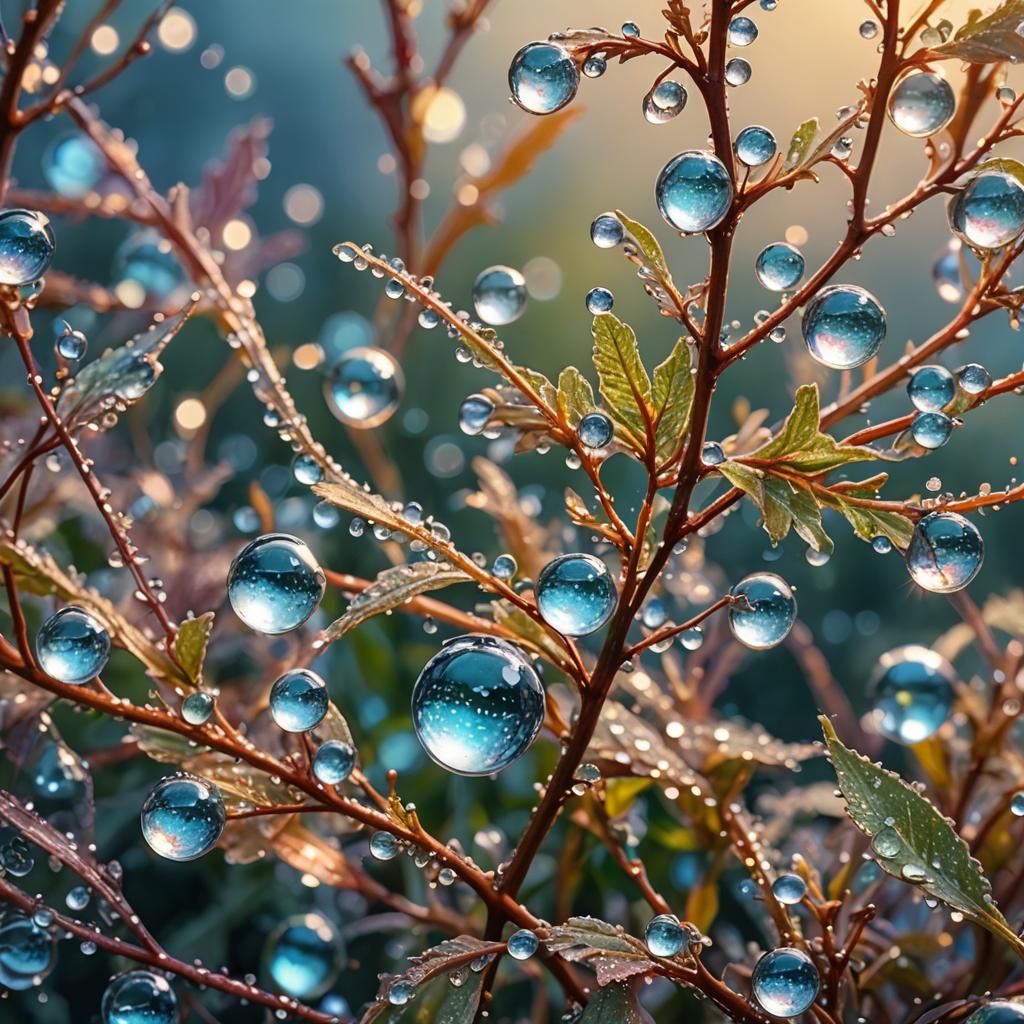The image presents an underwater scene, possibly digitally enhanced or artificially created, showcasing a cluster of small plants with thin, reddish-brown stems and an abundance of outstretching branches. These branches bear a mix of green leaves, some possessing a delicate, white fuzz. Scattered across the plants are numerous perfectly round, blue-tinged bubbles, varying in size from tiny to relatively large. The bubbles are highly reflective, adding a surreal touch to the image. The background is blurred, creating a depth effect that highlights additional plants and branches adorned with similar round bubbles. The overall color scheme features a dark blue backdrop with a gradient towards turquoise at the top, culminating in an orange glow in the upper right corner, suggesting an external light source. The meticulous arrangement of elements and the reflective quality of the bubbles give the scene an otherworldly, almost dreamlike appearance.